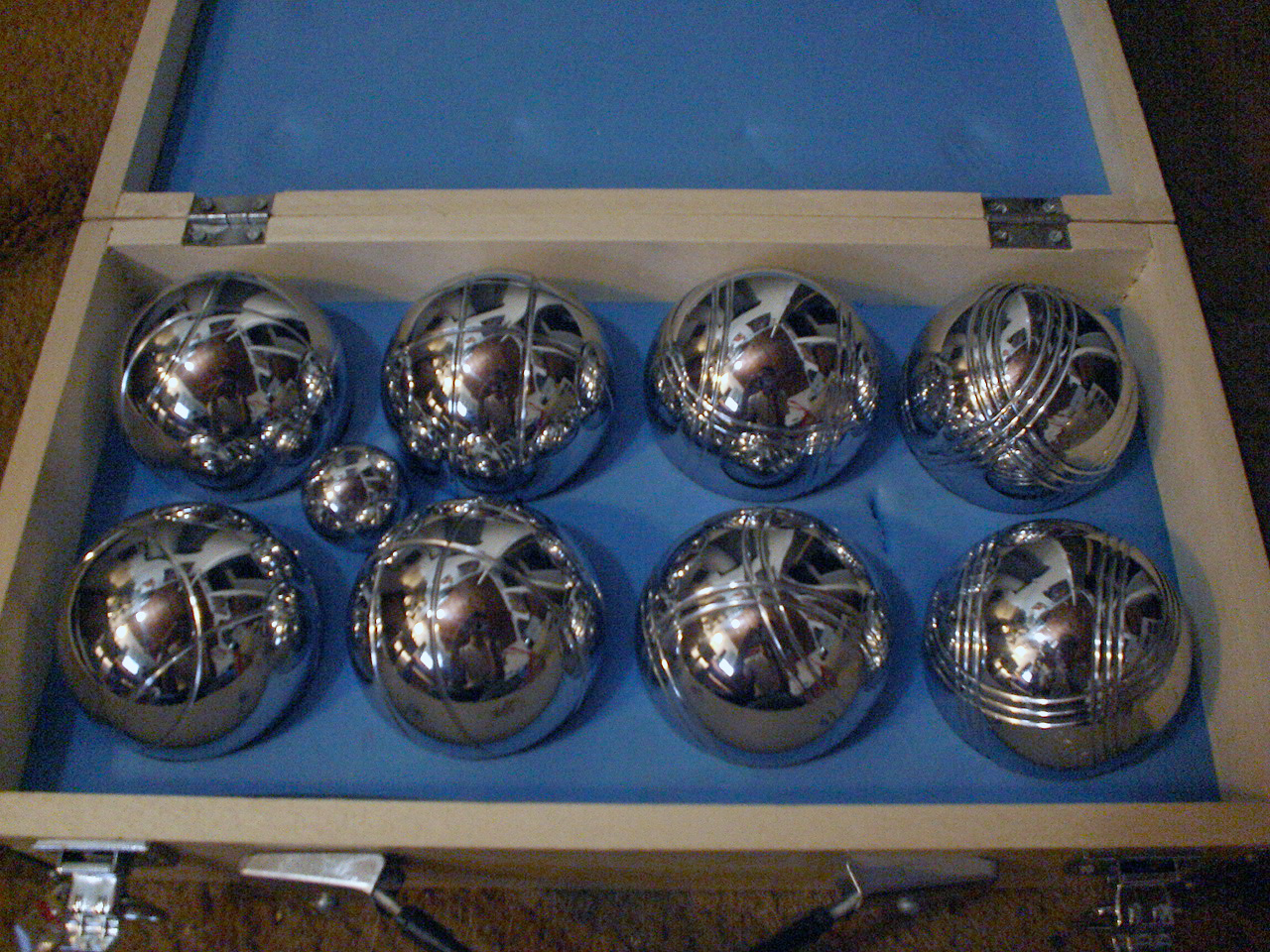This is a close-up of an opened wooden box, possibly made of light-colored maple wood with a grayish hue, sitting on light brown short carpeting. The box, finished with chrome hinges and latches, is lined with blue foam that snugly holds nine chrome-plated metal balls, mimicking the appearance of basketballs and soccer balls. Inside the box, there are eight larger balls and one smaller ball, with an indention suggesting space for a second small ball. A black leather handle, secured by chrome brackets, adorns the exterior. The highly reflective chrome balls capture the surroundings, including the person taking the photo and various objects on the room's walls.